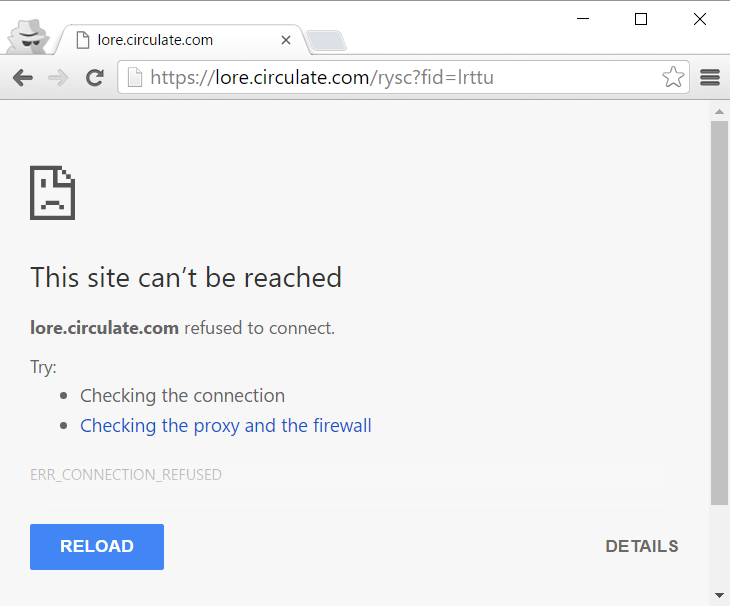In the image, a search engine page that cannot be reached is displayed prominently. The scene is a close-up of the browser window. Starting from the top left of the window, there are the standard control buttons: an 'X' for closing the window, a maximize button, and a minimize button. Adjacent to these controls, positioned on the left side of the top bar, is a logo featuring the silhouette of a man resembling a detective, complete with a trench coat collar, a classic brimmed hat, and sunglasses. The browser's tab indicates it is on the website "lore.circulate.com." The URL shown in the address bar is "lore.circulate.com/rysc?FID=LRTTU."